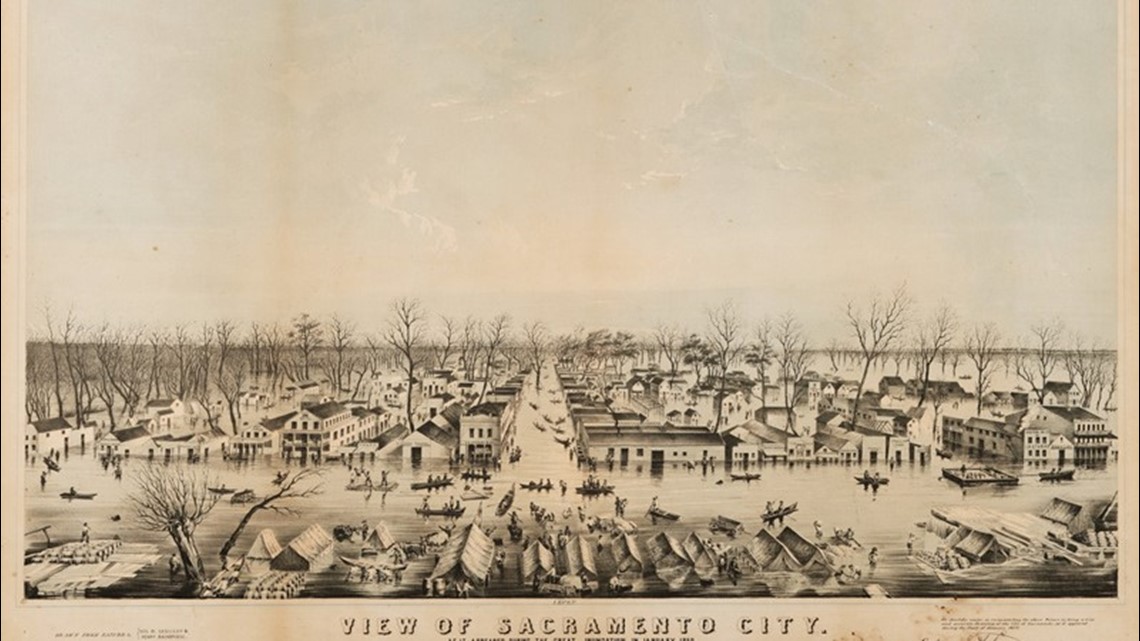This is an old, sepia-toned drawing on yellowed, brown paper, depicting a historical view of Sacramento City. The city, which appears to have been flooded, is devoid of traditional roads, replaced instead by waterways resembling those of Venice, Italy. The detailed scene shows multi-story houses and various buildings inundated with water, with the water level reaching up to the halfway mark of the first-floor doors. Small boats, manned by people, navigate the flooded streets, creating a bustling atmosphere. In the foreground, a shantytown comprised of tents, some with logs next to them and horses tethered nearby, hints at a temporary or make-shift settlement. The leafless trees scattered throughout the floodplain suggest it could either be winter or the result of environmental damage. The caption at the bottom of the image reads "View of Sacramento City," indicating that this drawing likely captures a significant historical moment, possibly a flood event, in California's capital city.